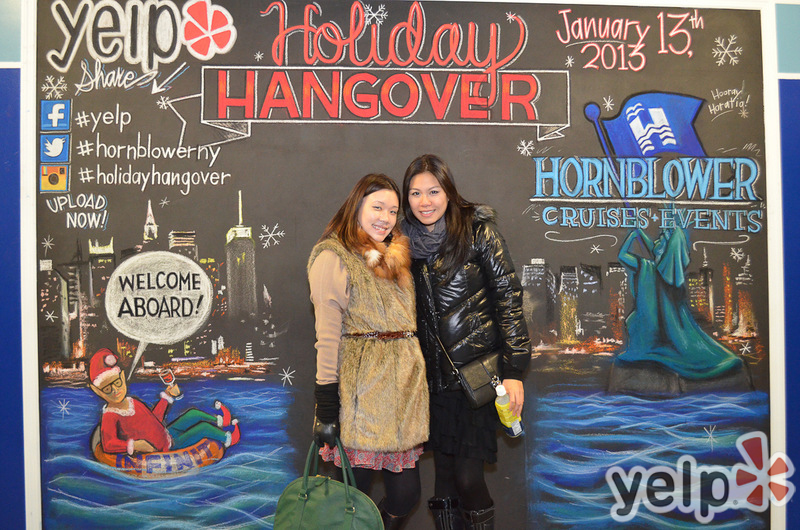In the photograph, two women of Asian descent are posing in front of a large, intricately decorated blackboard. The woman on the left is dressed in a stylish black puffer jacket, black boots, and a dark scarf, holding a bottle of lemonade in one hand. Her other arm is wrapped around her friend, who is dressed in a fur vest that reaches mid-thigh over outdoor wear, and is carrying a green purse. Both women are smiling warmly for the camera. Behind them, the blackboard is filled with detailed chalk art and writing. Prominently, in red letters, it says "Holiday Hangover." The blackboard also features a Yelp logo in the top left corner, with the date "January 13, 2013" in white on the upper right. Along the right side, the text "Hornblower Cruises Events" is visible beside an image resembling the Statue of Liberty blowing a horn, with a city skyline as the backdrop. On the left side, there's a whimsical drawing of an elf floating in a life preserver on blue water, adding to the festive and playful atmosphere of the scene.